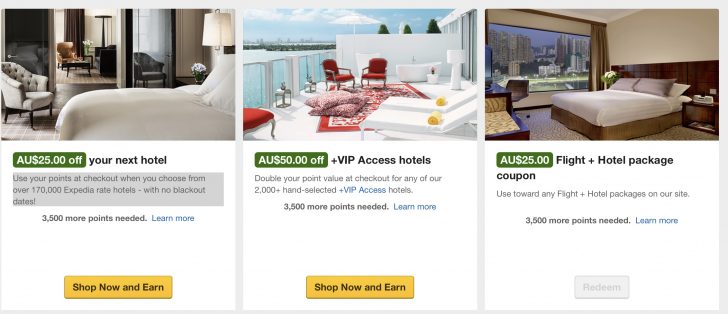Here is a detailed and cleaned-up caption for the given image:

---

The image showcases three different hotel room options with associated discounts and promotional details, possibly displayed on a travel booking platform.

1. **First Option**:
   - **Description**: The first hotel room shown appears to be set at night, featuring a predominantly gray color scheme.
   - **Discount**: Offers AUD 25 off on your next booking.
   - **Additional Information**: Includes a gray box with a promotional offer: "Use user points at checkout when you choose from over 170,000 Expedia rate hotels with no blackout dates. 3,500 more points needed. Learn more."
   - **Action Button**: A yellow button labeled "Shop now and earn."

2. **Second Option**:
   - **Description**: The second option highlights an outdoor balcony scene overlooking an ocean, predominantly decorated with red and white furniture.
   - **Discount**: Provides AUD 50 off and access to VIP hotels.
   - **Additional Information**: Including an offer to "Double your point value at checkout for any of the 2,000+ hand-picked VIP hotels. 3,500 more points needed. Learn more."
   - **Action Button**: A button saying "Shop now and earn."

3. **Third Option**:
   - **Description**: Depicts an interior view at night, showcasing a metropolitan skyline through large windows with decor featuring tan and brown tones.
   - **Discount**: Supplies an AUD 25 flight and hotel package coupon.
   - **Additional Information**: States: "Use toward any flight and hotel packages on our site. 3,500 more points needed. Learn more."
   - **Action Button**: The button is grayed out with the label "Redeem."

---

This caption provides a comprehensive and organized description of the visual and textual elements within the image.